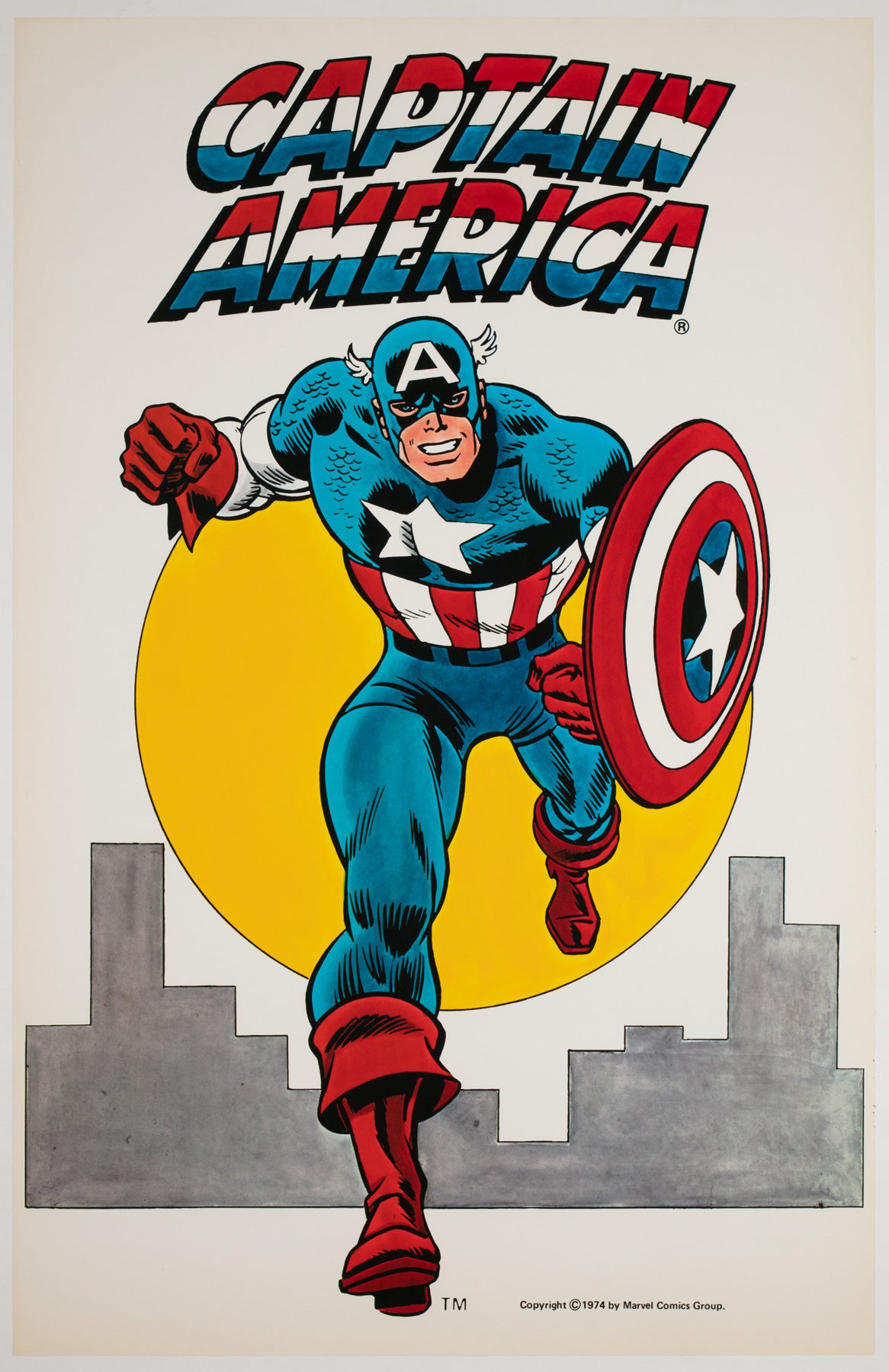This image depicts a vintage rendition of Captain America from 1974, prominently labeled "Captain America" in red, white, and blue striped lettering at the top. Captain America is illustrated in his classic blue uniform adorned with red and white stripes on his chest, a prominent white star, and a helmet featuring the letter "A" flanked by wings. He wields his iconic shield, which is similarly decorated with a white star at its center and red and white stripes encircling it, along with a hint of blue. He is pictured in an action pose, with one foot in the air and a fist raised, suggesting he is in mid-run. His costume is completed with red gloves and red boots. The background features a yellow-orange circle that may represent the Sun, and a simplified, grey city skyline composed of basic rectangular shapes, emphasizing its stylized, comic-book art form. At the bottom, there is a copyright statement: "1974 by Marvel Comics." The entire scene is set against a predominantly grey background, evoking a sense of nostalgia for the comic's golden age.